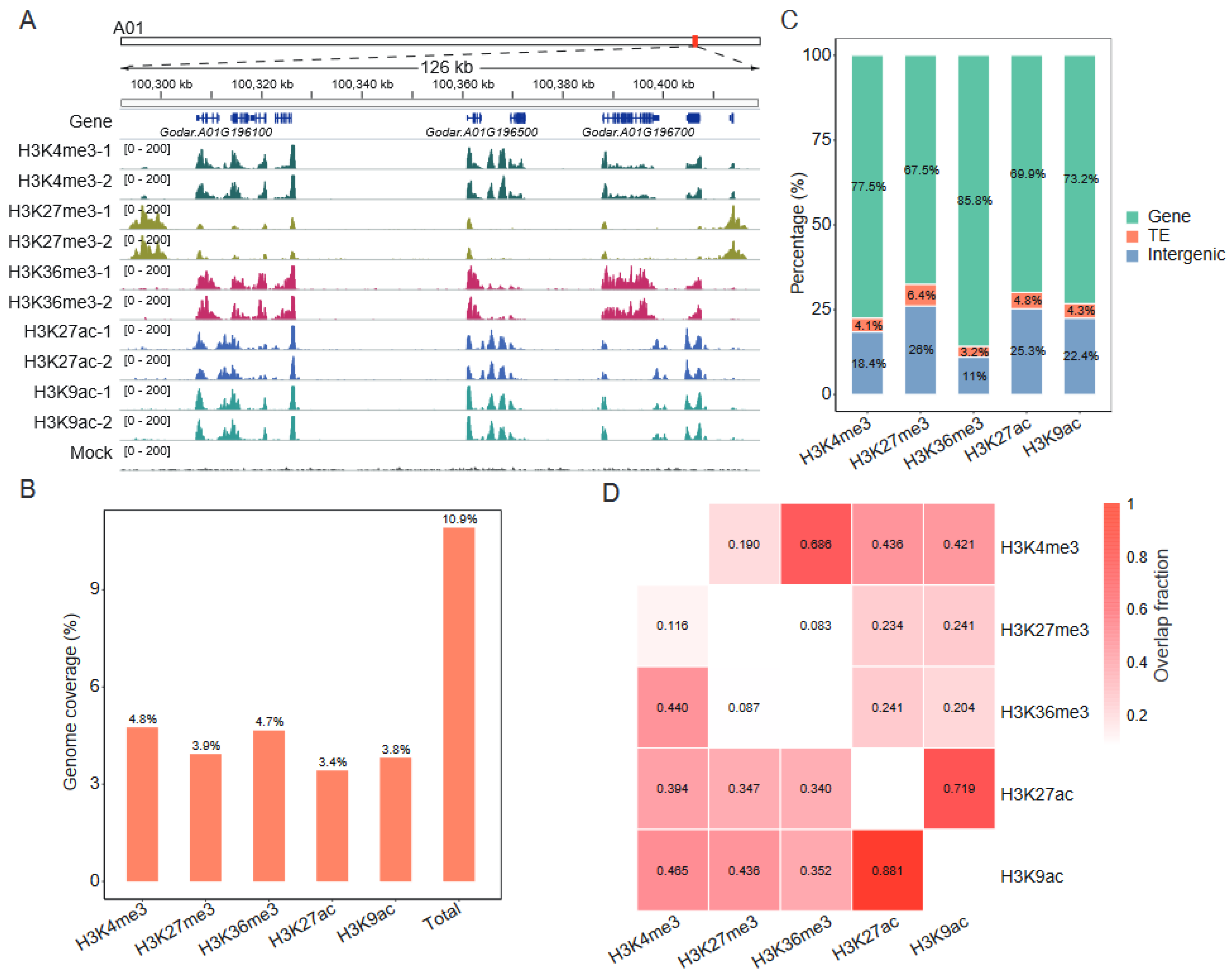The image is a scientific graphic composed of four different charts labeled A, B, C, and D, arranged in a 2x2 grid on a white background. Chart A appears to be a bar graph with labels such as gene, TE, and intergenic, implying a focus on DNA-related data. In Chart B, rectangular lines represent percentages like 4.8% and 4.7%, accumulating to a total of 10.9%, accompanied by various colors including green, light green, pink, and blue. Chart C uses color-coded rectangles—green for gene, orange for TE, and blue for intergenic—to show proportional data. Lastly, Chart D features a density or frequency diagram with red and white squares, indicating varying intensities within the dataset. Overall, the charts visualize complex genetic or scientific information with minimal textual explanation.